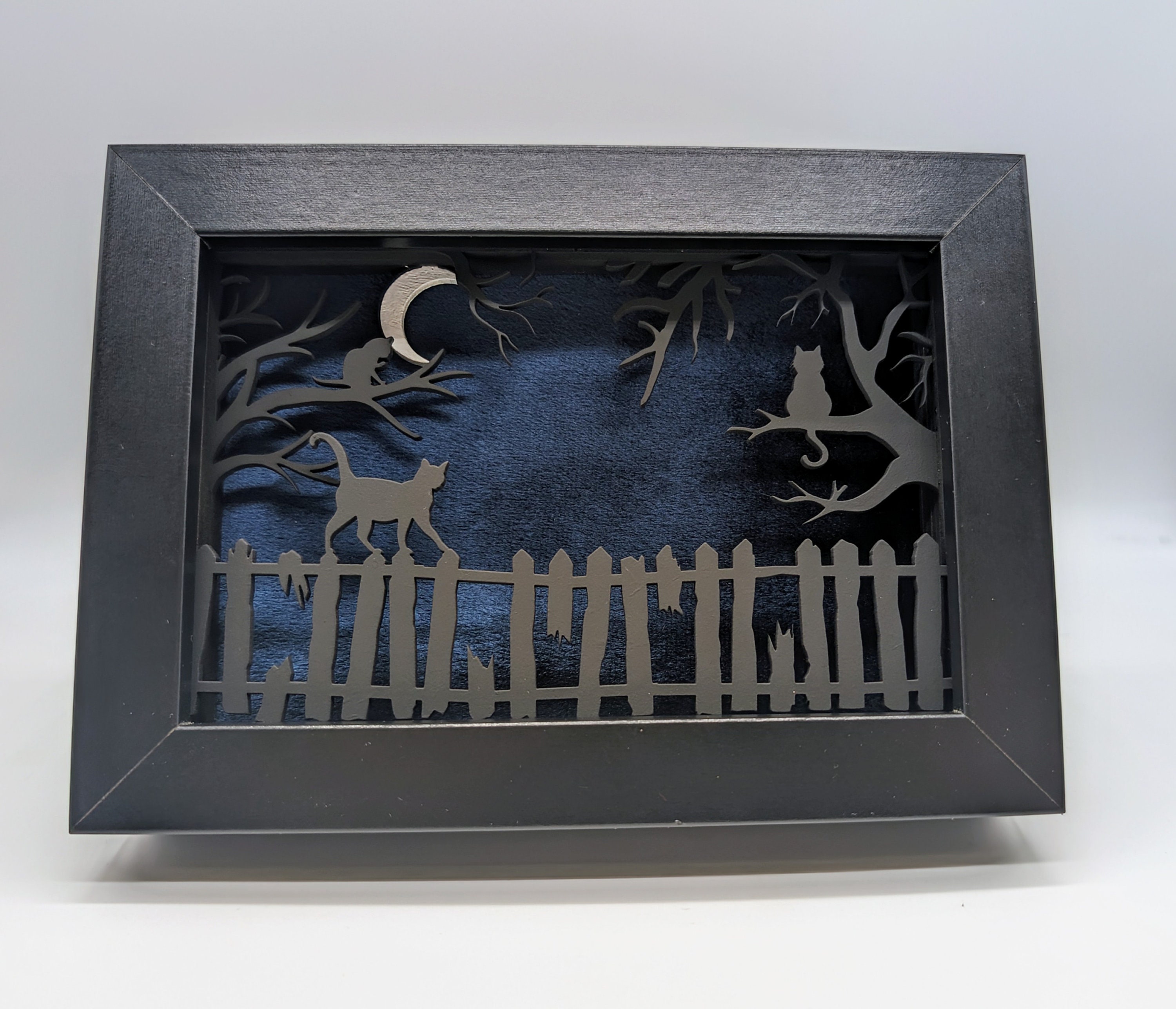This photograph captures a meticulously crafted shadow box artwork encased in a thick black rectangular frame. The interior features a luxurious deep blue velvet background, creating an enchanting night scene. The central focus of the piece is a series of multi-layered paper or metal cutouts that form silhouettes, giving the artwork depth and dimension. 

In the foreground, a silhouette of a cat gracefully walks on top of a broken picket fence, adding a sense of mystery. Flanking the fence are two trees, one on each side, with each tree's branches hosting a cat sitting serenely. Further branches stretch across the top of the shadow box, subtly contributing to the scene's depth amid intricate shadows. A prominent moon, cut out from a different material, casts a gentle glow from the left, partially obscured by one of the cats.

The blue velvet background, reminiscent of a starless night sky, enhances the goldish dark hue of the silhouette cutouts and contrasts with the bronzy black frame, which encloses this detailed, layered artwork. The shadow box is mounted on a white wall, angled slightly upward, showcasing its intricate detailing and dimensional composition.